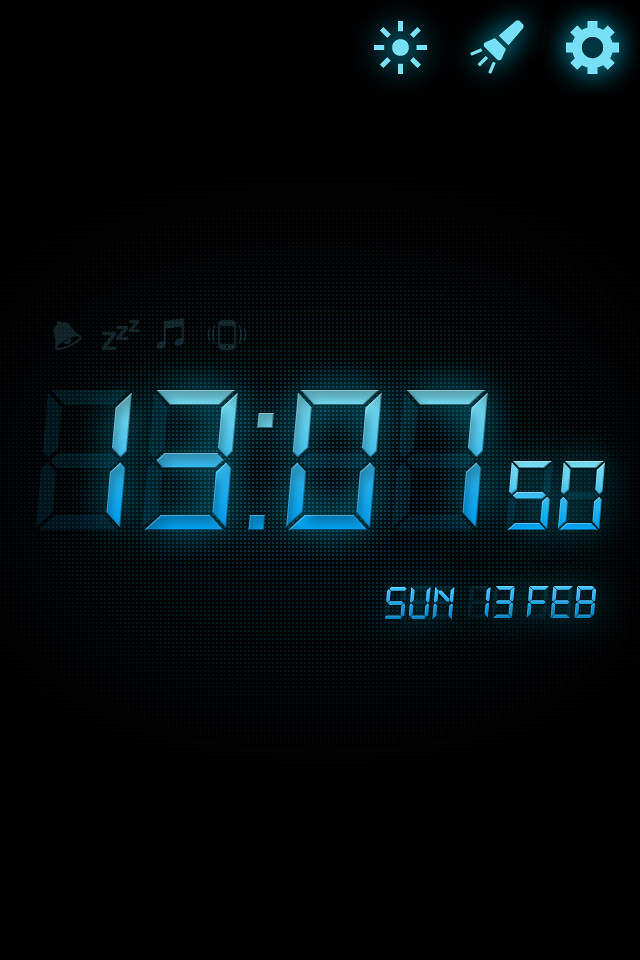The image showcases a digital clock with a striking neon blue display. On a completely black background, the time is prominently shown as "13:07" with "50" seconds. Below the time, to the right, the date is displayed as "Sunday 13 Feb," also in the same vivid turquoise hue. In the top right corner of the image, there are three brightly lit icons: a gear symbol, a flashlight, and a sun. To the top left of the main time display, there are grayed-out symbols of a bell, Zs, a music note, and a shaking phone. This suggests that the picture is a screenshot from a smartphone or similar digital device, emphasizing the sleek, minimalistic design and color scheme of the display.